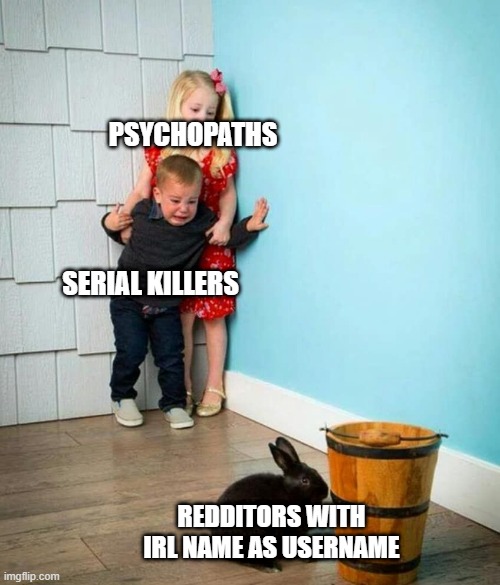Image Description: Meme Template Featuring Two Children and a Rabbit

In the image, two children stand in the corner of a room. The corner's left wall is a very light blue with a white baseboard, while the adjacent wall behind them has a white panel design with square and rectangular segments. The older child, a girl with long blonde hair tied with a pink bow, is wearing a red dress and golden shoes. She stands protectively behind a younger boy who appears frightened. The boy is dressed in blue jeans, light green shoes, and a dark shirt.

The girl has "psychopaths" written over her head, while the boy has the word "serial killers" over his. Both children are gazing down at a black rabbit at their feet. The rabbit is positioned next to a brown barrel with black stripes. Above the rabbit, the caption reads "redditors with IRL name as username."

In the very bottom left-hand corner of the image, the website "imgflip.com" is printed, indicating its source.